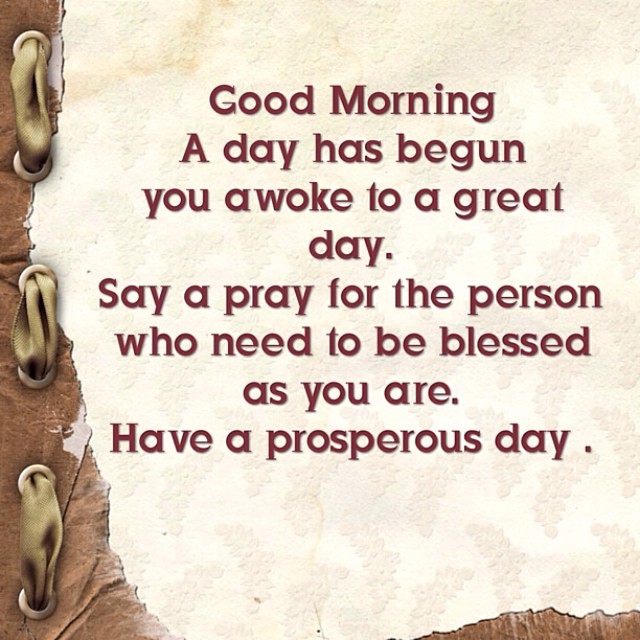The image features an inspirational graphic set against a beige backdrop that simulates the texture of old, worn parchment paper. The left side of this graphic is accentuated by a brownish texture, reminiscent of torn or burnt edges, and adorned with lace-like bindings that evoke the image of fabric threaded through eyelets. Centered on this textured background, the burgundy-colored text reads: "Good morning. A day has begun. You awoke to a great day. Say a prayer for the person who need to be blessed as you are. Have a prosperous day." The right side of the image remains lighter and cleaner, while the bottom right corner also features some of the brownish textural elements. The overall composition creates a harmonious blend of rustic charm and uplifting message.